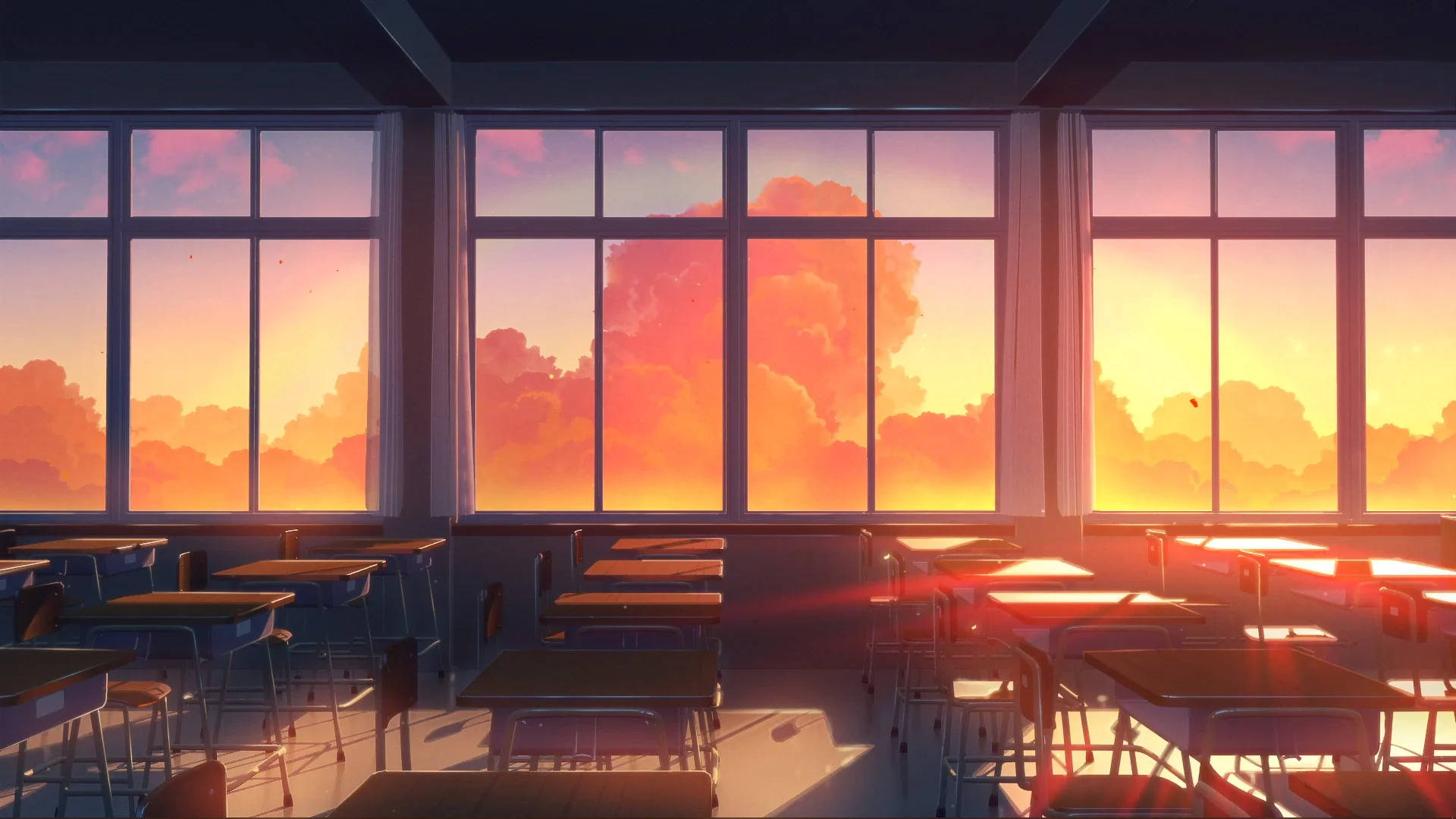The digital art illustration depicts a landscape-oriented image of an empty classroom. This classroom, occupying the lower third of the image, is meticulously arranged with rows of brown-topped desks, each supported by a silver base, and accompanying brown chairs, all positioned on a gray carpet. The desks and chairs are uniformly placed in perfect rows, their surfaces reflecting the vibrant colors streaming through the large windows at the back of the classroom.

The upper portion of the image showcases three expansive windows, a prominent central one flanked by two partially cropped side windows. Beyond the glass lies a dramatic, anime-inspired sky. The majestic sunset showcases a spectrum of colors—from the ghastly orange and yellow glow at the bottom to the rich purple and pink hues above. The scene outside is further dramatized by gray, puffy clouds, creating a surreal and almost apocalyptic atmosphere. The orange twilight enhances the indoor setting by casting warm light rays onto the empty desks, completing this vivid and evocative illustration.